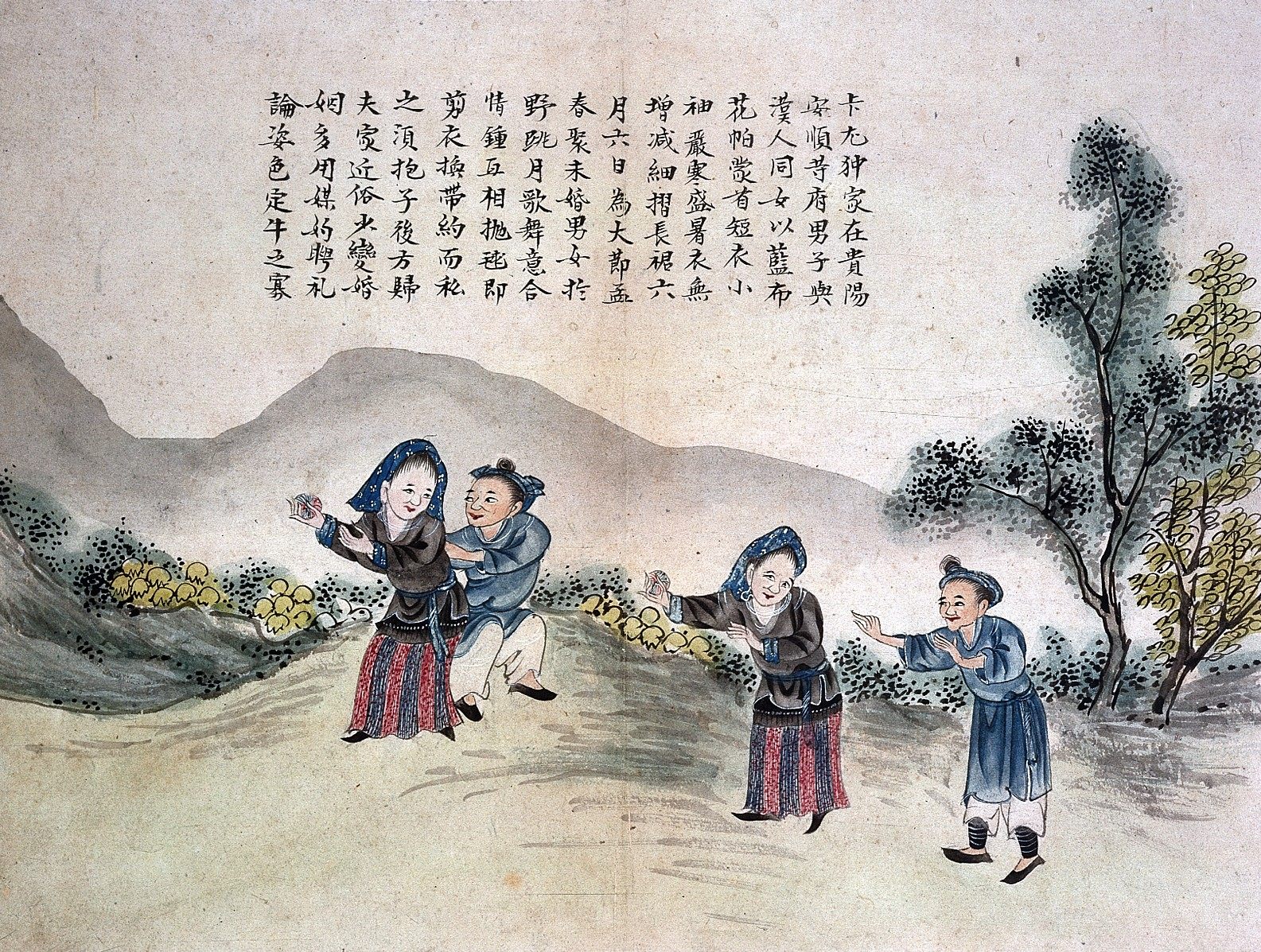The image appears to be a detailed, old painting or an illustration from a book, possibly from the early 20th century or even earlier. Set against a light gray background with gray mountains or hills, the scene displays seven lines of Asian text, written in straightforward calligraphy, likely in Chinese or Japanese kanji, cascading vertically down the left side of the image. The foreground features two sets of duplicated figures, a man and a woman, depicted in a sketch-like manner. The women have black hair draped with blue scarves and wear white tops paired with red and black striped gypsy skirts, while the men are attired in blue tunics and white pants. Central to the image, these figures appear to be dancing or positioned in a dynamic pose, set on a grassy hill. The image composition is horizontal and rectangular, suggestive of two pages from a book, and includes two trees on the right, one olive green and the other sage-colored, adding to the landscape’s classical charm.